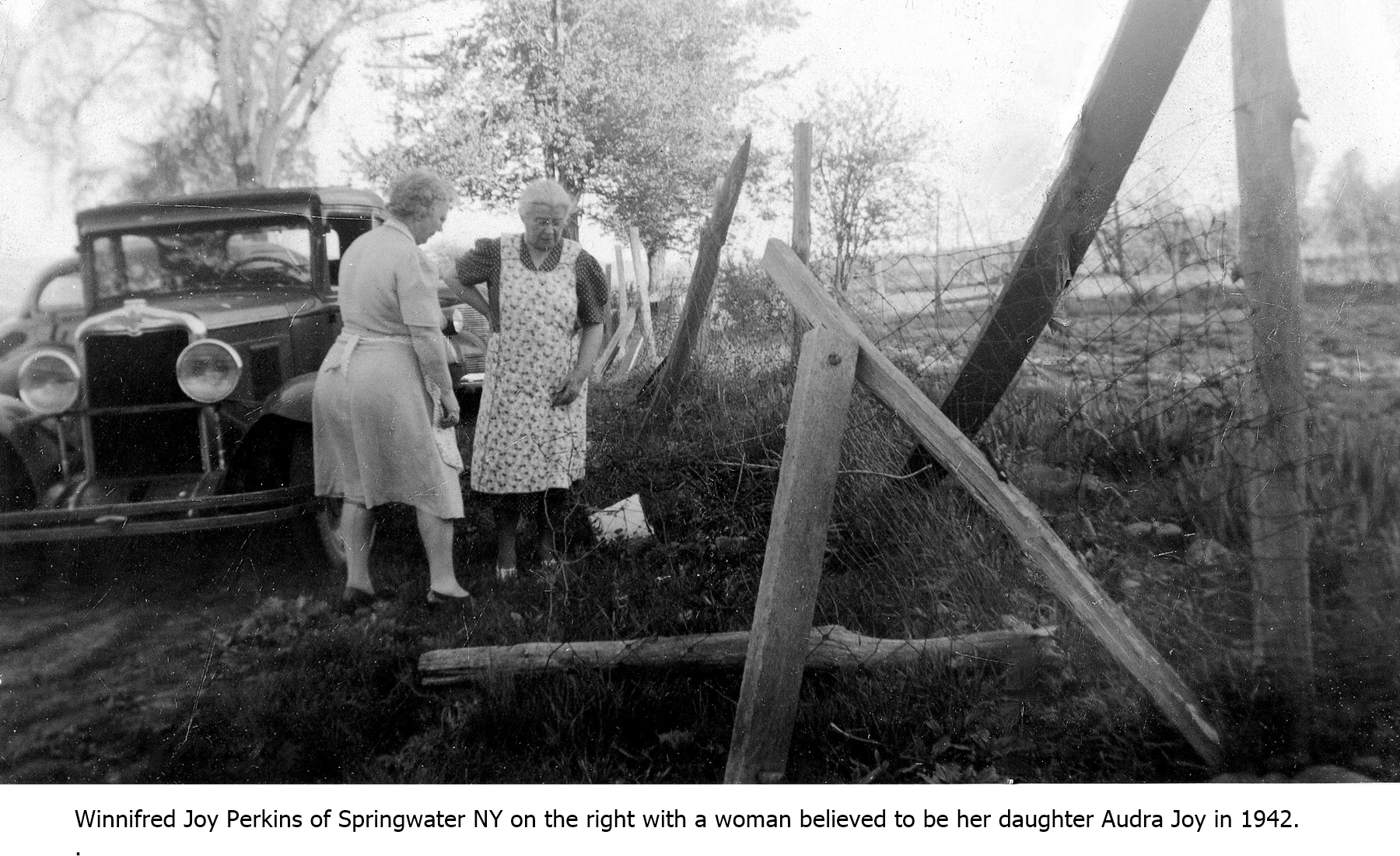In the black and white photograph dated 1942, two women are standing in front of a vintage early-1900s car, likely a Model T, characterized by its large headlights and substantial grille. The woman on the right, identified as Winifred Joy Perkins of Springwater, New York, is wearing a white dress and dark shoes, looking downward. Beside her and slightly in front, a woman believed to be her daughter, Audra Joy, is dressed in a polka dot dress with a floral printed apron. Both women have gray hair. They stand in front of a dilapidated wooden fence with scattered vertical and horizontal posts, some leaning or lying on the ground, possibly under repair. The scene is set against a backdrop of a distant field and tall trees under a bright, white daytime sky. The inscription at the bottom of the image clearly identifies the women and the year, providing a historical context to this evocative scene of rural life.